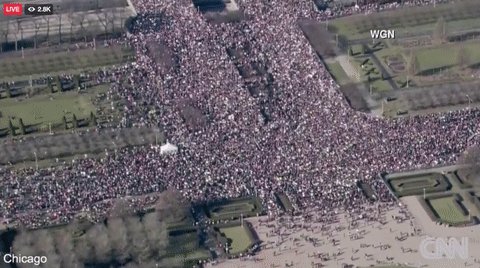The image depicts a high-resolution aerial view of an enormous crowd of people, captured as a screenshot from a live news broadcast. Presented in a rectangular format with a 2:1 aspect ratio, the photograph is marked by text overlays providing additional context: in the bottom right corner, semi-transparent grey text reads "CNN"; in the bottom left corner, white printed text states "Chicago"; while the top right corner has the letters "WGN" prominently displayed. The top left corner features a small red rectangle with "LIVE" written inside it in white text, adjacent to a black rectangle with "2.8K" in white text.

The scene shows a sea of people densely packed along a road surrounded by greenery, suggesting a large public gathering such as a concert or rally. The crowd is so vast and densely packed that individual details of the people are indistinguishable, with individuals appearing as mere dots of various colors, including white, grey, and black. The setting includes landscaped areas and possibly a large public garden, with grid-like patterns of green patches and shrubs visible around the concrete surface where the crowd is situated.

The elevated vantage point offers a broad, comprehensive overview, emphasizing the sheer scale of the gathering and contributing to an impression of mass and movement, as some people are seen spilling outwards from the central congregation area.